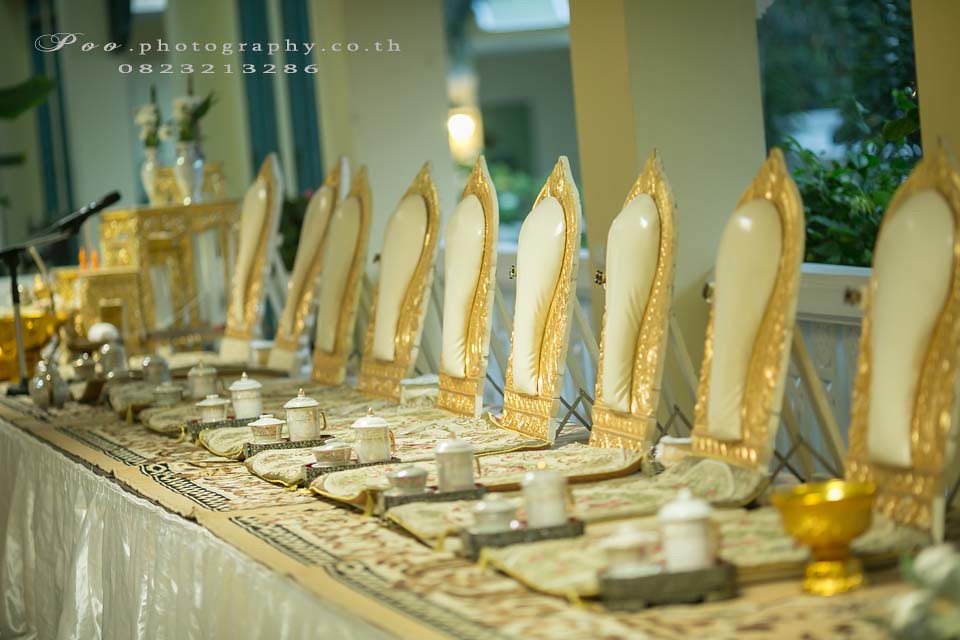This photograph captures a meticulously arranged dinner scene inside a refined, well-lit room with large windows flanked by concrete posts. At the center, a long table is draped in a pristine white cloth with an intricate gold-trimmed mat running across its surface. Each place setting features a delicate arrangement of white teacups, tiny teapots on tiny trays, and gold-rimmed cream cups, all aligned with precision. Surrounding the table are cream and gold chairs with high, slender backs and gold outer frames. The chairs are upholstered in cream fabric, providing a luxurious touch.

In the background, a gold table adorned with flowers is visible, adding to the room's elegant ambiance. Majestic golden ornaments and statues stand against a white backdrop, further enhancing the opulent setting. A black microphone angled diagonally suggests the photo was taken during a seminar or conference. Details such as green bushes and trees, along with a white structure seen through the windows, hint at an inviting outdoor view. The image is watermarked with "poophotography.co.th" and a contact number, adding a professional touch to the scene.